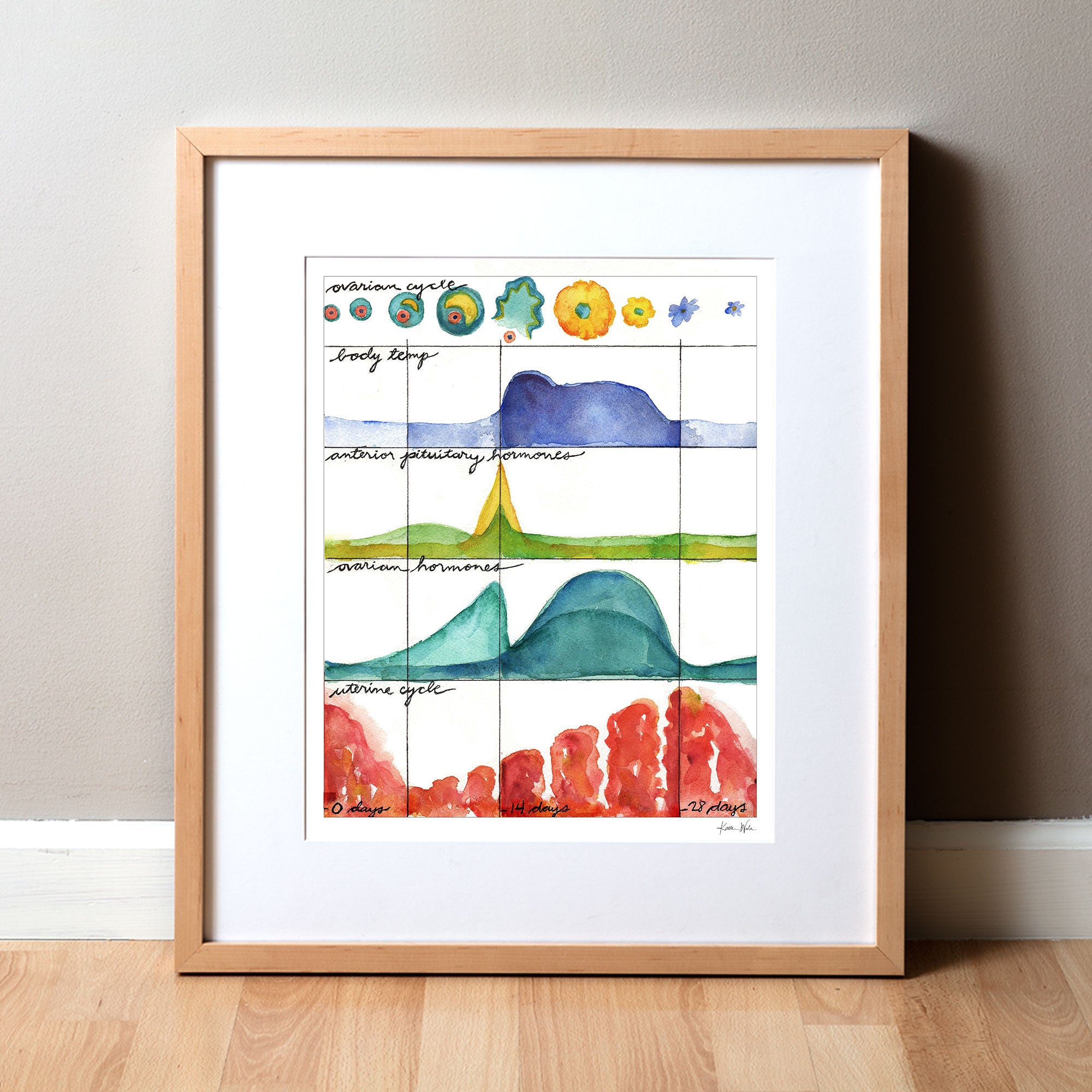The image depicts a framed watercolor painting resting on a light-colored wooden floor, leaning against a gray wall. The frame is made of light-colored wood, complemented by a white inner border. This scientific artwork is divided into distinct sections, each providing detailed visual information on various aspects of the female reproductive cycle. 

At the top left corner, the painting is labeled "Ovarian Cycle," featuring a series of progressively larger green and pink circles with black dots at their centers, eventually forming tree-like and floral shapes. Below this, a section labeled "Body Temp" presents a blue graph depicting fluctuations in body temperature.

Further down, there is a segment titled "Anterior Pituitary Hormones," highlighted by three graphs—two green and one yellow, with the yellow graph peaking higher than the others. Adjacent to this is the "Ovarian Hormones" section, marked by three distinct blue peaks.

Towards the bottom, the "Uterine Cycle" is portrayed with a red graph that initially dips from a high point, then rises again. The timeline across the entire painting is demarcated at intervals of zero days, 14 days, and 28 days. A small artist's signature can be seen in the lower right-hand corner, adding a personal touch to the detailed scientific illustration.